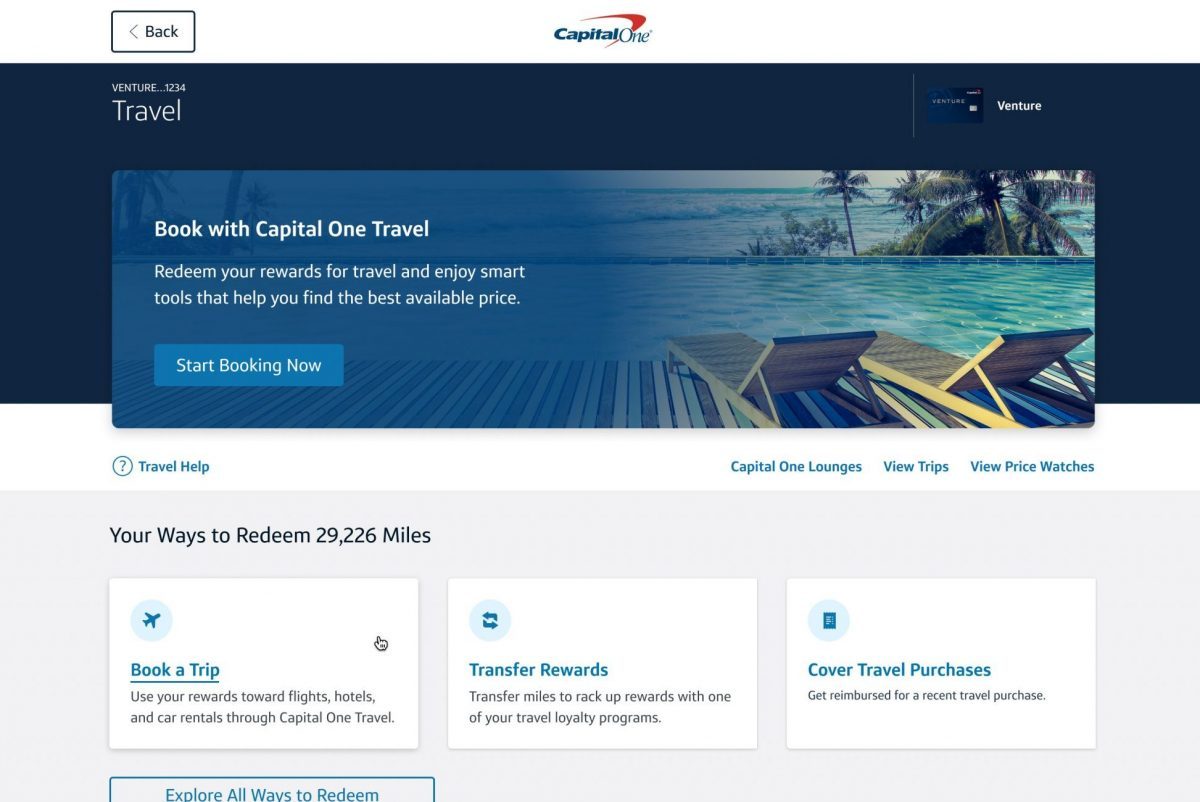The image displays a promotional ad from Capital One Travel, featuring various elements aimed at enticing customers to use their rewards for travel-related benefits. 

At the top-left corner, an arrow within a rectangle pointing to the left signifies a navigation option to return to the previous page. The headline reads, "Travel, Adventure..." followed by an intriguing "One, Two, Three, Four," setting the tone for an exploration theme.

The main text promotes the usage of Capital One Travel, urging users to "Book with Capital One Travel." It highlights that customers can "Redeem your rewards for travel and enjoy smart tools to help you find the best available price." A call-to-action button, "Start Booking Now," is prominently displayed in a blue rectangle.

Additional features outlined in the image include:

- "Capital One Lounges"
- "View Trips"
- "View Price Watches"
- "Travel Help," indicated by a circle with a question mark.

The section "Your Ways to Redeem 29,226 Miles" is emphasized, showcasing three white rectangles that detail the options:

1. **Book a Trip**: Use rewards towards flights, hotels, and car rentals through Capital One Travel.
2. **Transfer Rewards**: Transfer miles to rack up rewards with one of your travel loyalty programs.
3. **Cover Travel Purchases**: Get reimbursed for recent travel purchases.

Finally, another blue rectangle at the bottom encourages users to "Explore All Ways to Redeem."

This well-organized promotional visual promotes various ways clients can leverage their travel rewards, emphasizing convenience and flexibility.